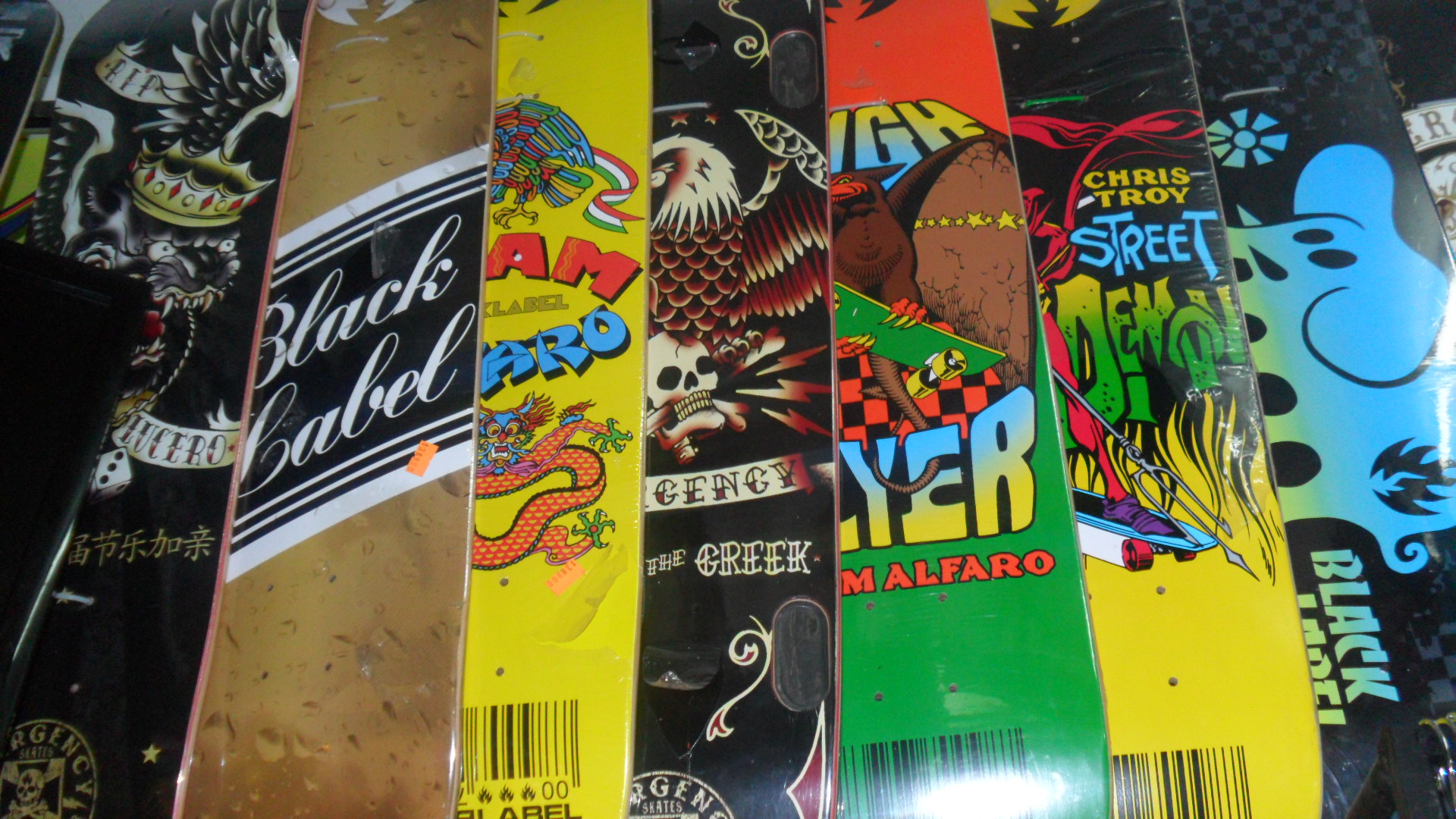The image is a close-up view of what appears to be the bottoms of nine skateboards or snowboards, displayed side by side in overlapping fashion. The intricate and vivid artwork on each board ranges from monstrous creatures to stylized text. Starting from the left, the first board features a flying monster wearing a crown. Adjacent to it, the second board displays the text "Black Label" in a curly white font against a black background. The third board presents a dragon accompanied by a bird on a yellow background, embellished with red, white, and green ribbons. The fourth board showcases an eagle standing on a skull with partially visible text that includes "the Greek". Following that, the fifth board has a large bat with a long tail on a red and green backdrop. The sixth features a demon riding a skateboard against a black and yellow background with text that reads "Chris Troy Street Demon". The seventh board has a melting, ball-like blue creature. While the eighth board, which is only partially visible, contains some form of vintage tattoo-like art potentially involving a strange tiger or dragon with text that could include Japanese or Spanish words. All these boards feature unique, elaborately painted designs, capturing a spectrum of artistic styles and themes.